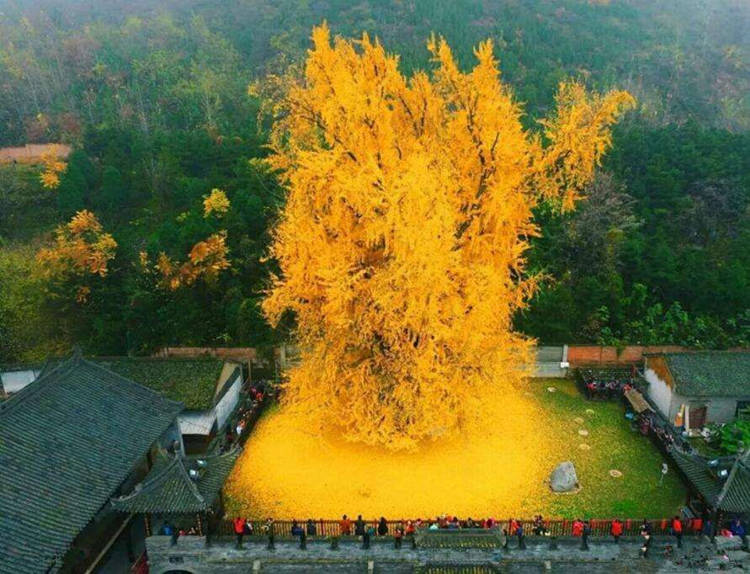The image features a towering, vibrant yellow ginkgo tree positioned in the center of a square garden, possibly situated atop an Asian-style architectural structure. The ginkgo’s brilliant yellow and bronze leaves blanket the ground beneath it in a thick, circular layer, indicating it is fall. The courtyard garden where the tree stands is bordered by a fence railing, behind which around 20 people are gathered, intently observing the magnificent tree. The courtyard itself has green grass interspersed with stones. Surrounding the courtyard, in the background of the photograph, is a landscape of trees showing hints of green and yellow, hinting at the transition to autumn. A mountain can also be seen in the distance, adding to the picturesque setting.